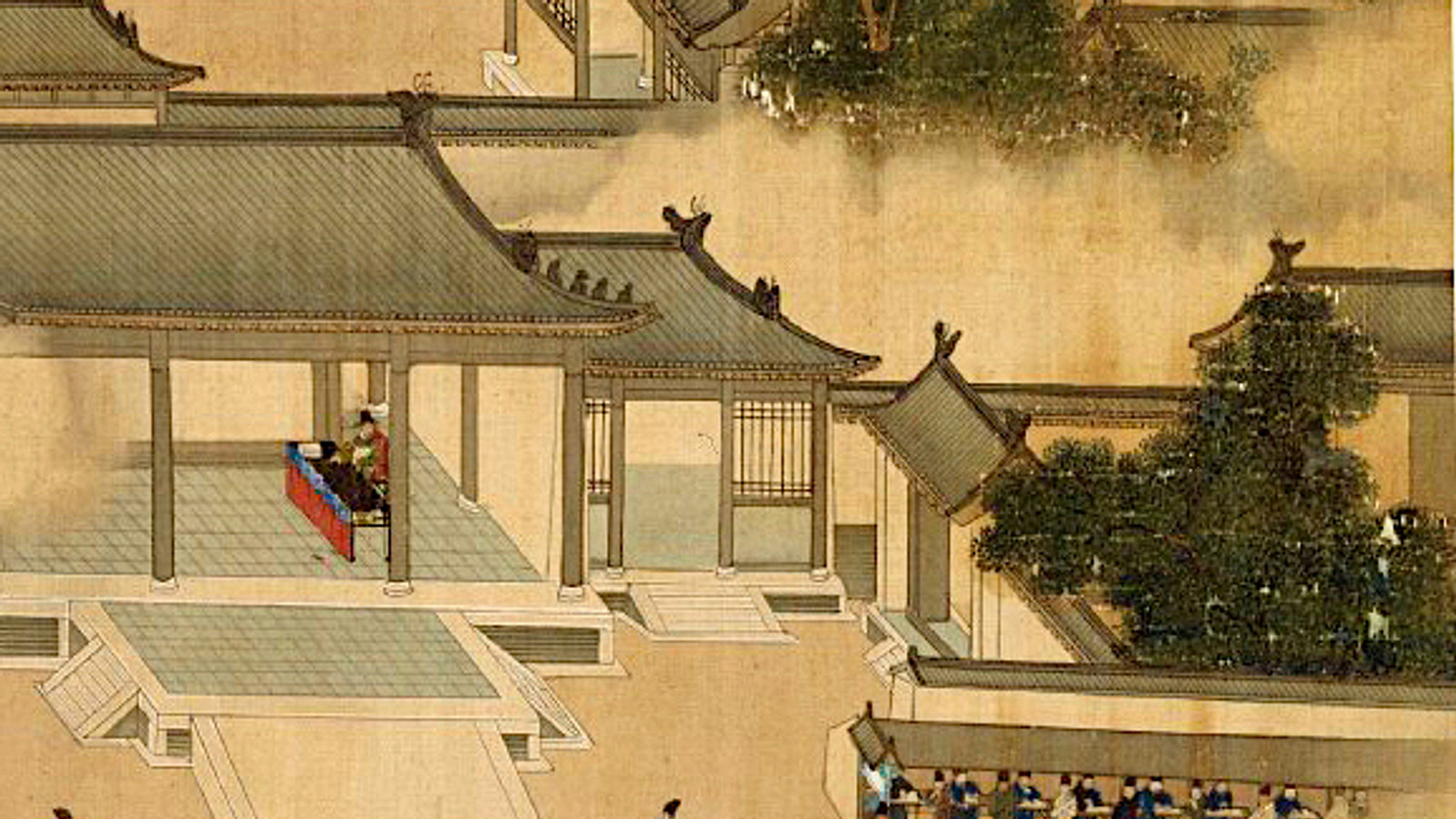This detailed image depicts an ancient Chinese scene reminiscent of historical paintings. Dominated by faded tones of yellow, green, black, red, blue, and white, the setting features several traditional Chinese architectural structures with characteristic sloping roofs that flare at the corners. 

Prominently, on the left side of the painting, a man is seated behind a table within one of these structures, distinguished by a purple top, blue sides, and red bottom. In contrast, the bottom right corner reveals a classroom scene where multiple children are studying under the supervision of a teacher, all within a similarly designed school building. The intricate details include a courtyard enveloped in white fog, nestled between two trees, adding to the serene and somewhat mystical atmosphere. Additionally, some blurriness at the top right suggests more buildings and tree-like structures, contributing to the painting's depth and historical ambiance. No text is visible in the image, further emphasizing the visual storytelling through its artistic elements.